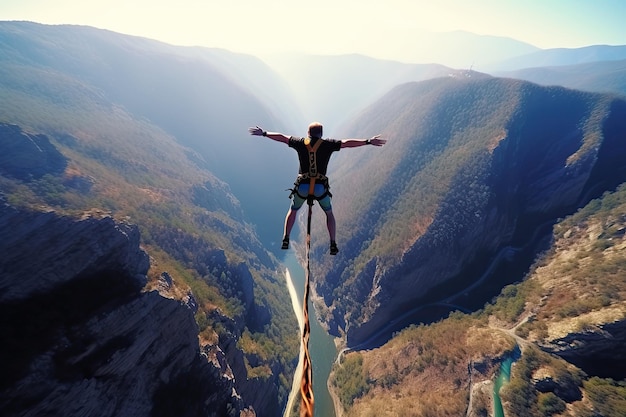In this detailed image, we see a man in midair, seemingly in the midst of a thrilling bungee jump. He is suspended by a tannish brown bungee cord that extends from a structure likely high above, possibly a bridge. The man is depicted splayed out with his arms outstretched and legs straight down, wearing a black shirt, green and blue shorts, white gloves with black wrists, and black shoes. An orange, black, and white harness marked with the number 34 secures him. 

The backdrop is a breathtaking natural landscape featuring high-elevation hills and rock formations on both sides, which are covered in green and yellowish bushes, plants, and trees. The rocky terrains display a mix of white, gray, tan, and black hues. At the base of the valley, a river winds through, running greenish-blue in color and providing a lush contrast against the rugged environment. The sky above is primarily white with patches of blue, illuminating the entire scene and highlighting the dramatic descent of the bungee jumper.